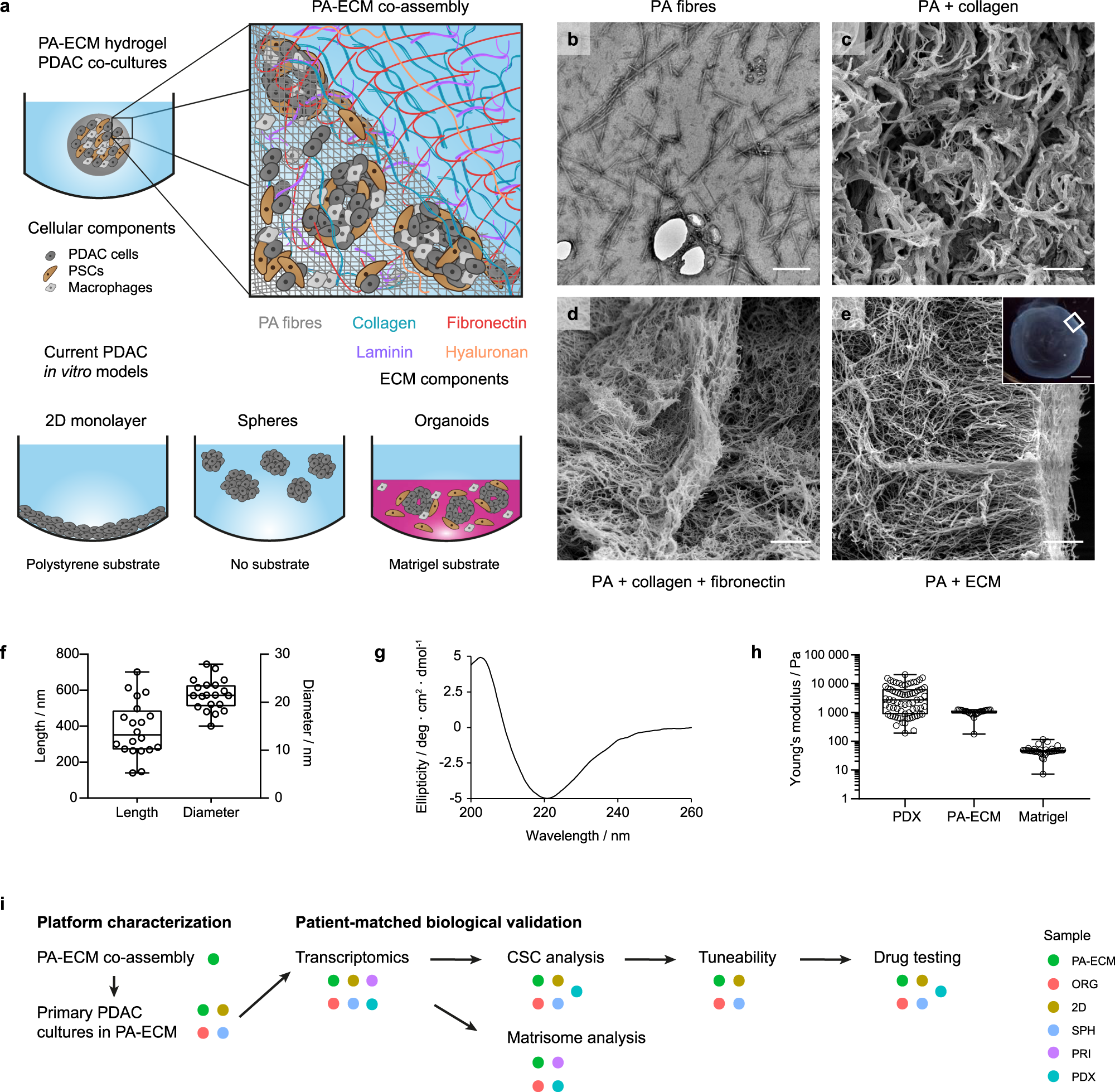The image presented is a detailed and complex multicolored scientific poster set against a white background, focusing on advanced research topics. The poster is divided into various sections, each containing a mix of digital graphics, x-ray or microscope images, and graphs. The upper left corner features drawings and text discussing PA-ECM hydrogel PDAC co-cultures, while the top right corner includes four black and white panels labeled as PA fibers, PA plus collagen, PA plus collagen plus fibronectin, and PA plus ECM. The central area displays multiple images and charts denoted by the letters A through I. The lower section of the poster contains a series of graphs, some color-coded, and a labeled section with colored dots. The data is organized under headings like "platform characterization" and "patient-matched biological validation," showcasing spheres and organoids and emphasizing the scientific complexity of the research presented.